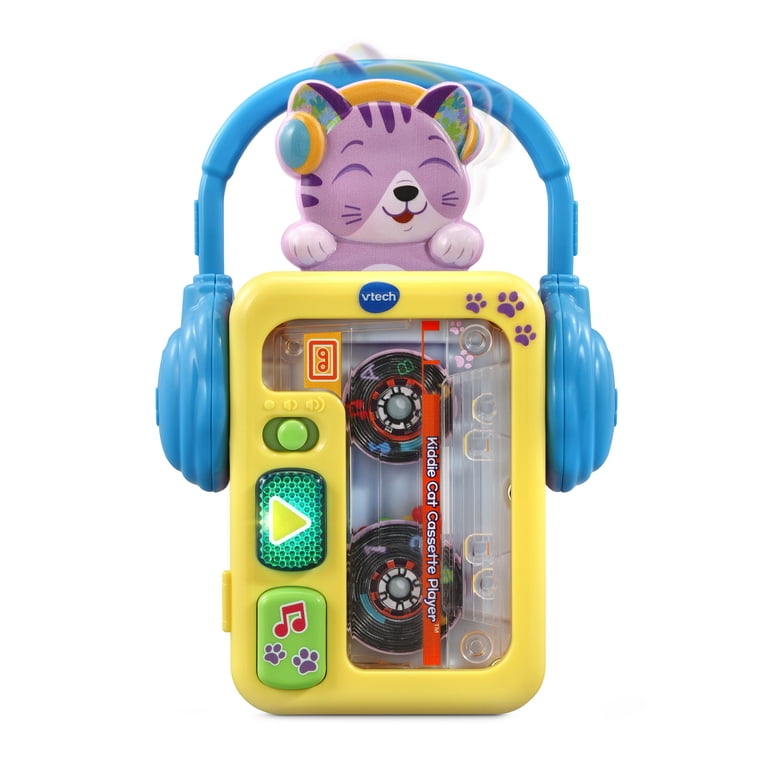The picture features a vibrant children's toy reminiscent of a classic cassette player, manufactured by VTech. The main body of the toy is a cheerful yellow with prominent green buttons. In the center, there is a transparent window revealing round black reels where a tape would play. The toy has a lit green play button marked with a yellow triangle, and nearby, another green button adorned with a musical note and paw prints. A sliding green button on the side serves as a volume control, allowing for sound adjustments.

At the top of the toy, a cat figure sits happily. This purple kitty cat has closed eyes and a serene smile, donning orange headphones with blue ear pieces. The toy's branding is prominently displayed with white text that reads "VTech" at the top and "Kitty Cat Cassette Player" on a red strip below the clear window.

Additionally, the cassette player includes chunky, blue, plastic headphones attached to either side. The toy is detailed with purple cat paws and other charming feline features, emphasizing its playful design. This delightful toy captures the nostalgic appeal of vintage cassette players while adding a whimsical, child-friendly twist.